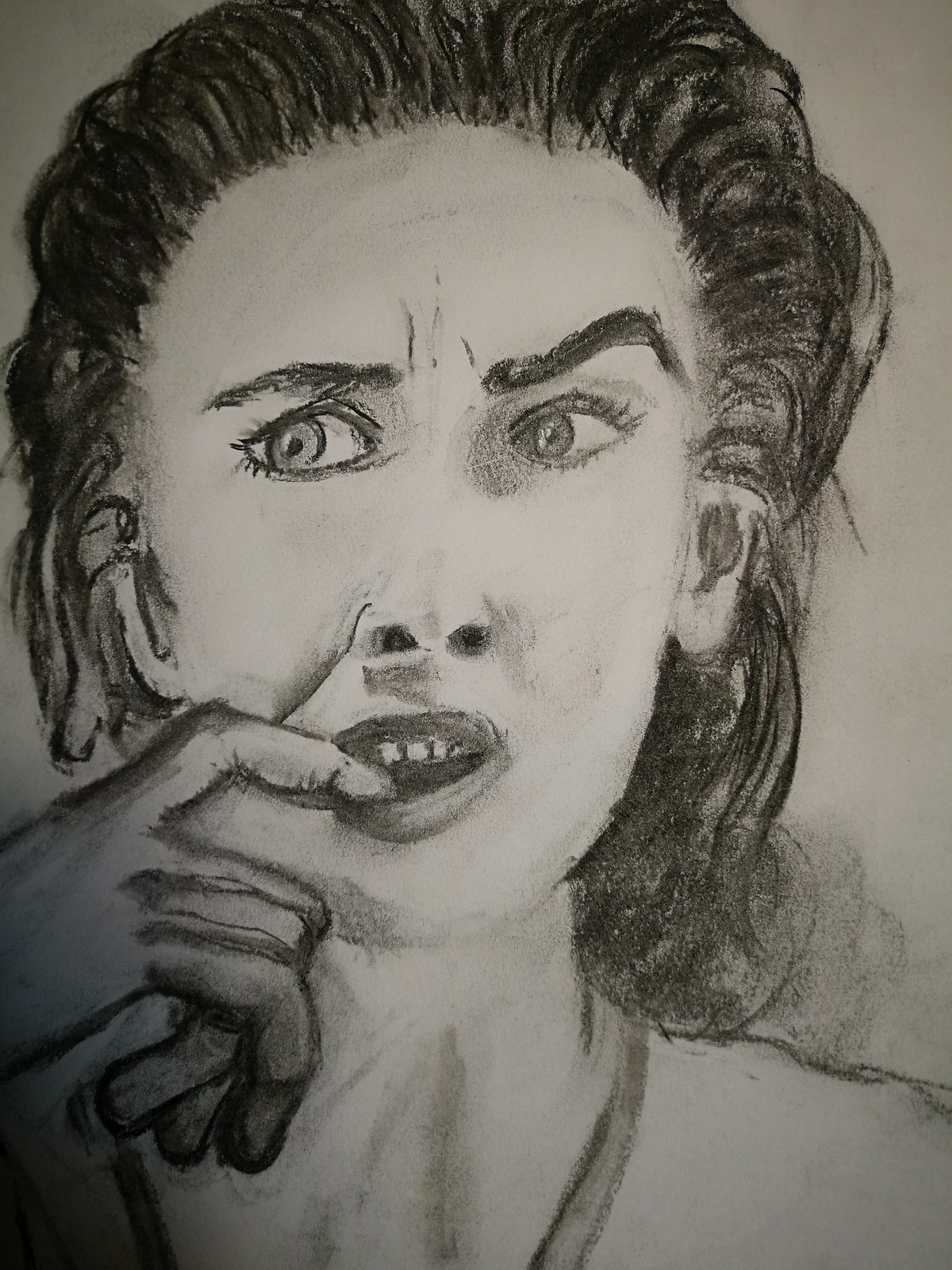This charcoal drawing portrays the face and shoulders of a woman, capturing a vivid expression of fear or confusion. Her black hair is neatly combed back from her forehead, accentuating her arched left eyebrow. She gazes toward her right, focusing on something beyond the frame. Her mouth is slightly open, and her right hand hovers near her lips, with her index finger delicately inserted between her parted lips. Around her neck, there is a visible necklace or the outline of her shirt, adding depth to her portrayal. The background is accentuated with shadows cast by her hair, creating a dramatic effect. Notably, her right hand's fingers appear disproportionate, mirroring the slight asymmetry in her frontally depicted face, where her misaligned eyes gaze sideways. The imperfections in the proportions add a unique, haunting quality to the overall composition.